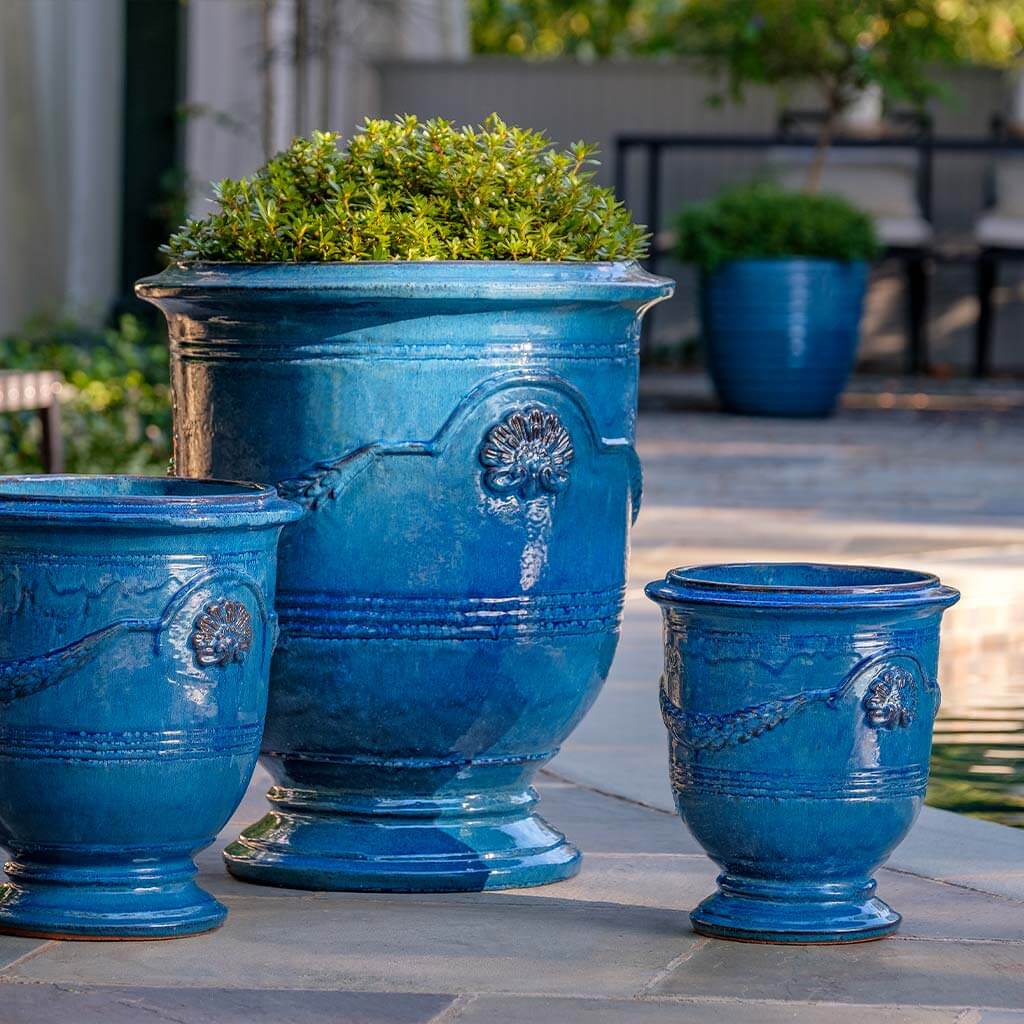The image is a vibrant color photograph set in a seemingly urban, outdoor tiled area, possibly part of a plant store or gardening center. The foreground prominently features three aesthetically crafted blue vases. The middle vase, the tallest among the three, contains lush green plants and is designed with elegant lines and details, including a crest resembling a peacock with an arched line and wreath motif. The smaller vase on the right and the medium-sized vase on the left are both empty. In the blurred background, another large blue vase, which is not flared at the bottom, also contains plant material. The setting suggests it is daytime, and the grayish tiles beneath the vases enhance the vibrant blue hues. Sparse trees and a wall, perhaps the edge of a bench, are subtly visible in the background, completing the serene yet urban ambiance.